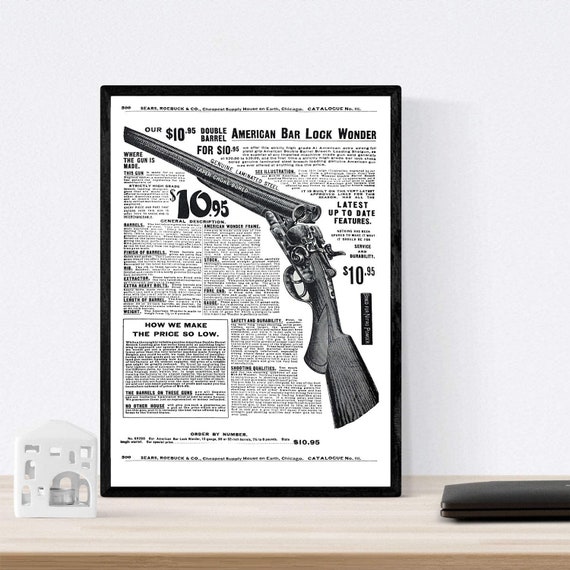The image showcases a detailed photograph of a framed, old newspaper advertisement for a shotgun. The black-framed ad is centrally positioned on a light gray tabletop, with a thin brown edge visible at the very bottom. On the left of the tabletop, a small white object, possibly an adapter, can be seen, while a thin black case is partially visible on the right edge.

The advertisement itself is for the "American Bar Lock Wonder" double-barrel shotgun, priced at $10.95. The ad is printed on white paper with prominent black writing that highlights key details. The text at the top says "R1095 Double Barrel American Bar Lock Wonder," followed by "$10.95" beneath it. The featured image of the shotgun runs diagonally from the upper left to the bottom right, showcasing the gun half-cocked with an open barrel. To the right of the gun image, there's small black print detailing its latest features.

A large "1095" is printed prominently to the left of the gun image, and below it, a white box contains bold black text reading "how we make the price so low," accompanied by a descriptive paragraph. Additional small black text and paragraphs provide more details about the shotgun, including its latest features and price justification. The ad sits near a gray laptop against what appears to be a gray wall, emphasizing the vintage appeal of the artifact.